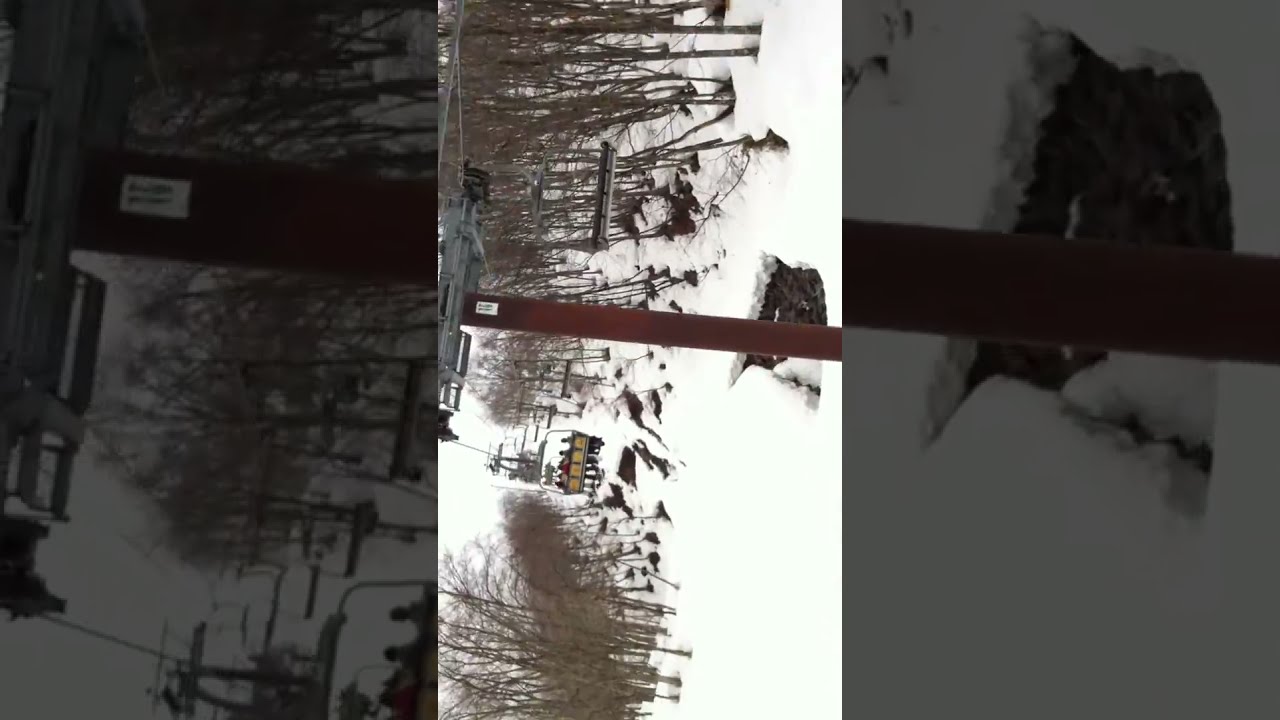This photograph, rotated 90 degrees to the left, captures a snow-covered mountainside dotted with barren, brown trees. At first glance, the image appears bordered by vertical black strips on both sides, framing the central scene. The sky above the mountain is a bright, almost blinding white, suggesting a sunlit afternoon. A busy ski resort atmosphere is depicted by a yellow ski lift running horizontally across the top of the image, with some seats occupied by people and others left empty. Each ski lift bench, designed to hold four people, is suspended by a wire and moves up and down the slope. The dynamic and slightly offbeat perspective, combined with the vivid contrast of white snow, barren trees, and bright yellow lifts, creates a striking portrayal of an active winter day on the mountain.